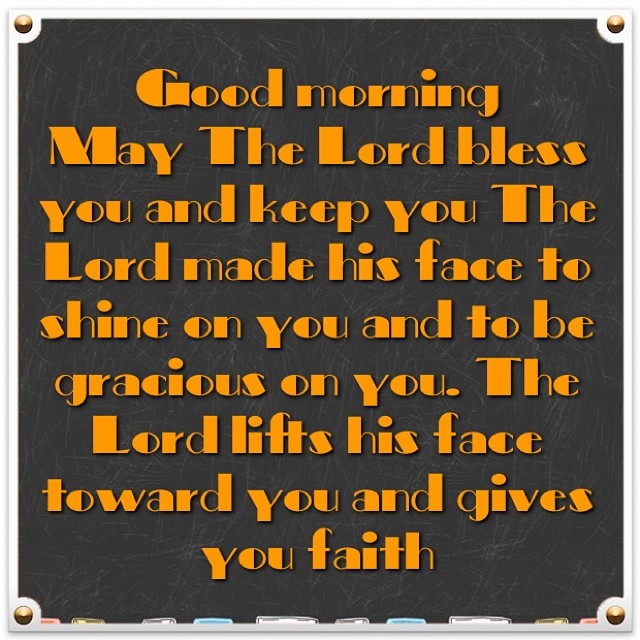The image is a photograph of a plaque that appears metal, with four rivets—one in each corner. The background has a dark, gray-brown hue reminiscent of a chalkboard, accented by scratch-like markings and white framing around the edges. In the corners, there are gold-yellow round dots. At the bottom, on top of the white frame, are small rectangular shapes in red, yellow, white, and blue, resembling chalk or markers. The text, in bright orange font, reads: "Good Morning. May the Lord bless you and keep you. The Lord make His face to shine on you and be gracious to you. The Lord lift His face toward you and give you peace."